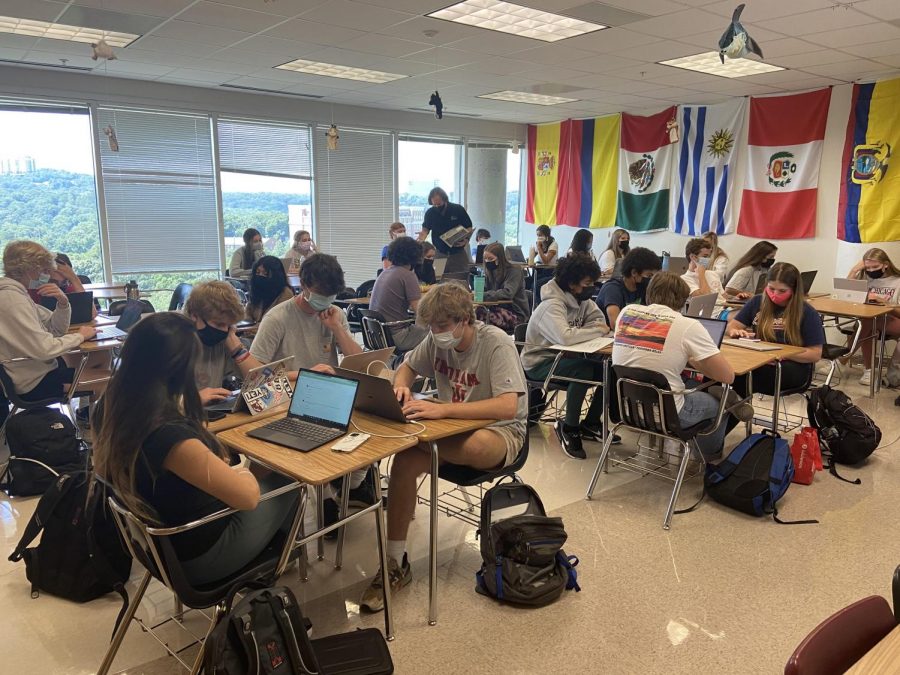This daytime color photograph captures a bustling classroom filled with approximately 20 masked teenagers, each seated at desks equipped with laptops. The students have their desks arranged in clusters, fostering interactive group work. The white-tiled floor is littered with backpacks of various colors, predominantly black and blue, with at least one red bag in sight. The room is well-lit by natural light streaming through five windows, some of which are partially open, revealing glimpses of green trees and nearby buildings outside.

The walls are adorned with flags from six different countries, adding a multicultural flair to the learning environment. One older man in a white shirt sits at a desk, while a woman—presumably a teacher—moves around the room, handing out materials and engaging with students. The orderly yet dynamic atmosphere reflects a modern classroom setting where safety measures, like face masks, are diligently observed, and the mix of natural light and educational decor creates an inviting space for learning.